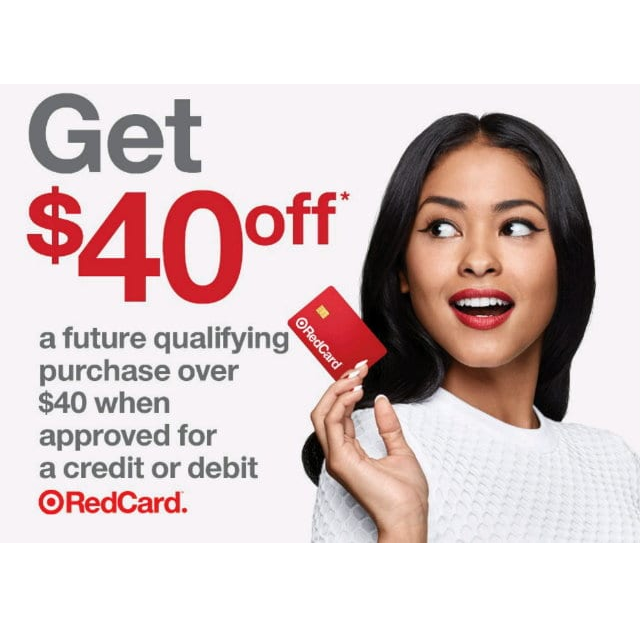This advertisement showcases a special promotional offer, enticing new applicants to apply for a Red Card, whether it be a credit or debit option. The offer promises a $40 discount on a future purchase of $40 or more, once the application for the Red Card is approved. The visually appealing design highlights the significant savings potential for prospective cardholders, emphasizing the ease and benefits of obtaining the Red Card. The advertisement aims to attract customers by offering them substantial savings on their future purchases after successfully acquiring the Red Card.